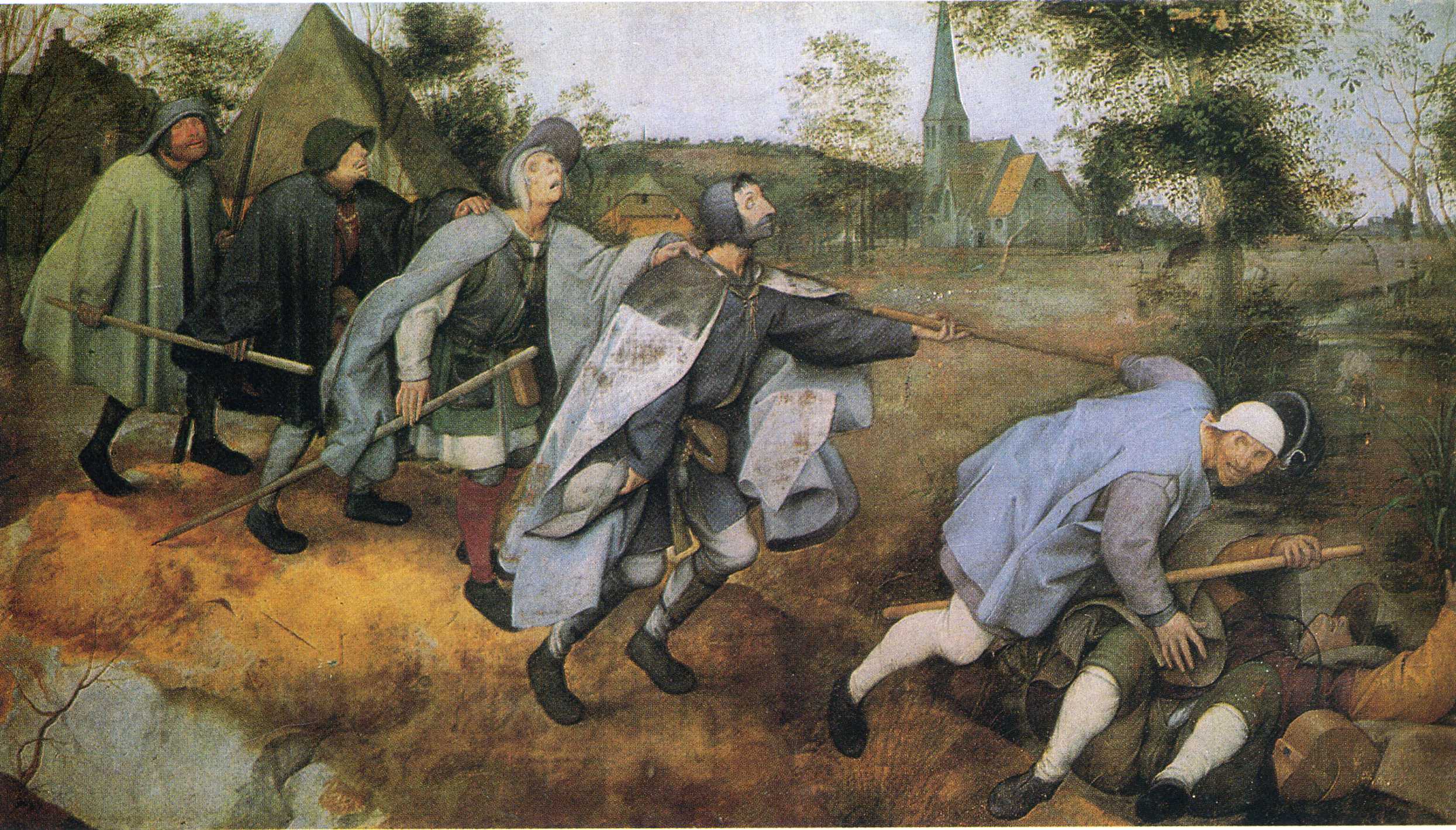This horizontally aligned rectangular painting depicts a historical scene set under a grayish-white sky. At the top of the painting, a white-stone building with a brown roof and steeple, likely a cathedral, stands in the background. To the left of the building, a couple of brown tents are visible, and a tall, narrow-trunked tree with green splotches of leaves occupies the upper right portion. 

In the foreground, six men appear to be in the midst of a battle, possibly under attack, arranged in a line along a grassy bank. They are wearing long capes in shades of gray and black, and military helmets reminiscent of those from the 1300s. The men carry wooden poles: two men at the back, a woman and a man in the middle, and another man in front of her all holding these sticks. 

The man closest to the viewer on the lower right is lying on his back with his knees bent, seemingly injured, clutching a wooden pole. The man in front of him, dressed in a blue coat, is bending over, perhaps in a protective stance, while also holding onto a stick that both he and another man behind him are grasping. The four men at the back are all looking upwards, while the second man in line glances to his right, his eyes shifted in an almost backward glance towards his comrades. The scene is set against a rustic, brushy foreground adding to the historical ambiance of the painting.